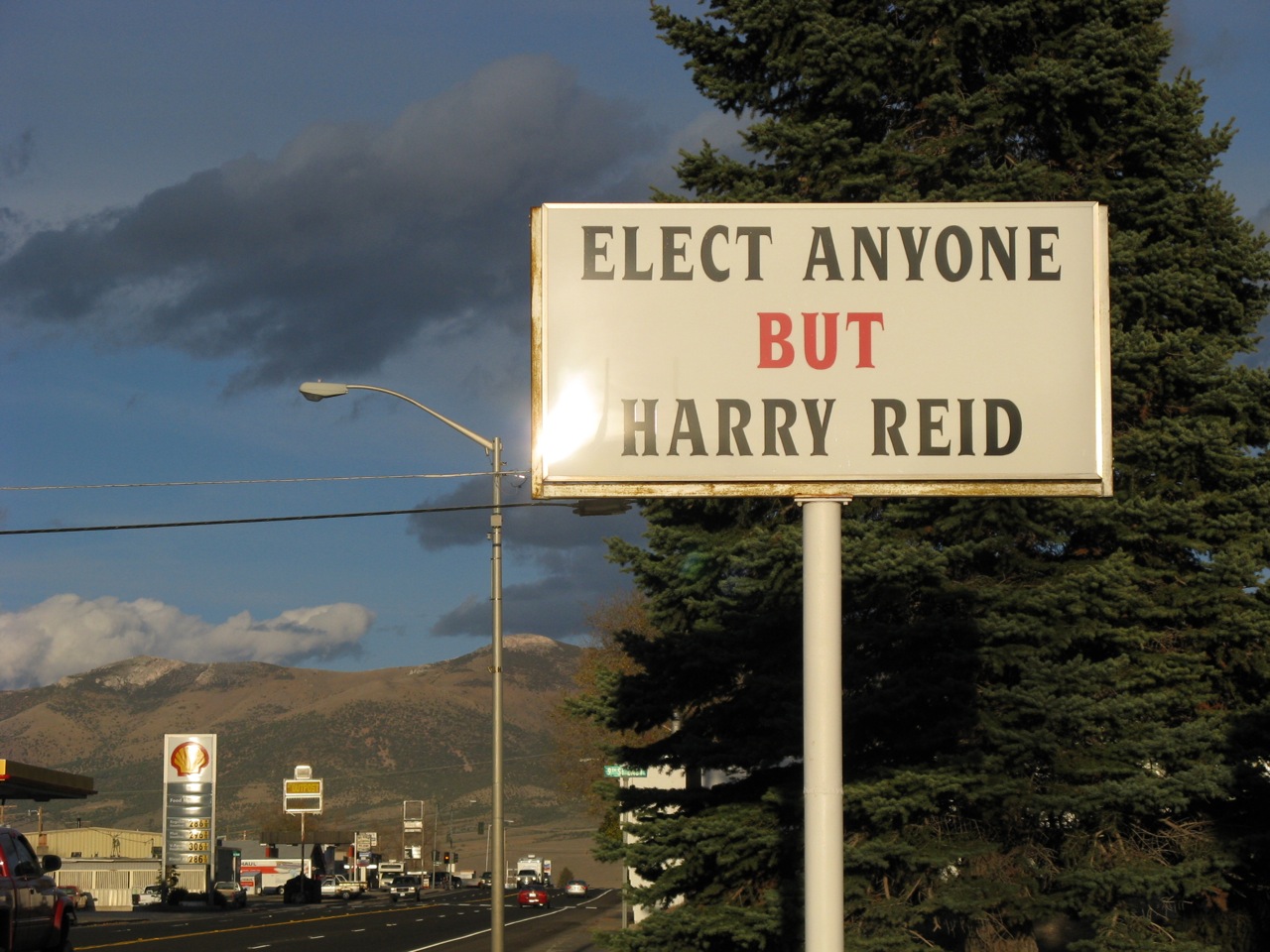This close-up photograph captures a white, rusted metal sign mounted on a white pole, prominently reading "elect anyone but Harry Reid" in black and red letters. A sun glare touches the bottom left-hand corner of the sign, and the edges show visible rusting, particularly on the bottom and left-hand side. Behind the sign stands a tall evergreen tree. To the left, there's a bustling retail area featuring a reflective Shell Gasoline sign, distinguished by its yellow and red colors. The background reveals a road leading towards distant mountains with cars and trucks travelling. Above, the sky is a mix of blue with both white and dark gray clouds, adding depth and contrast to the scene.